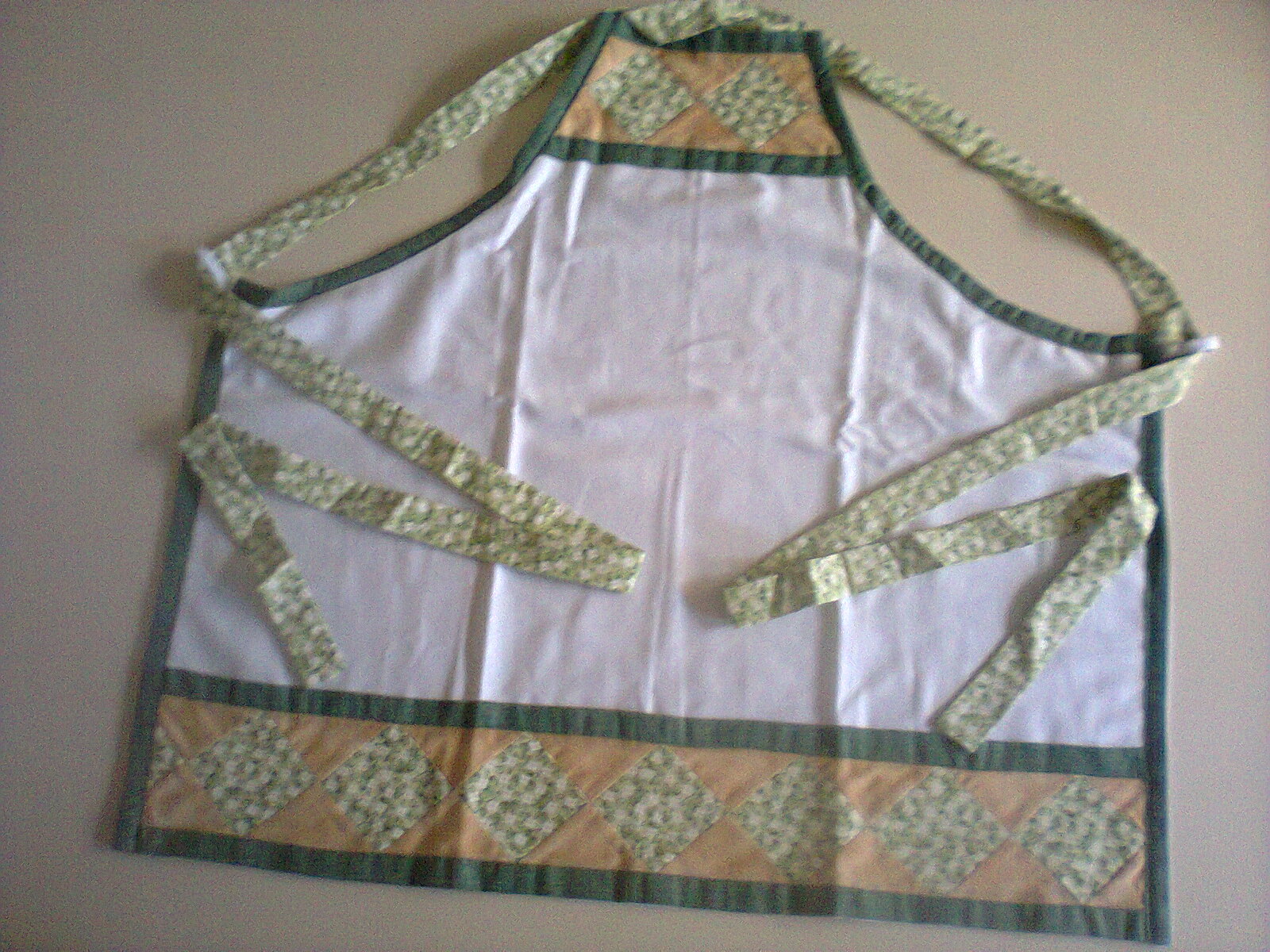This photograph features a homemade, quilted apron laid out on a smooth, white surface. The apron is primarily white with a thin, dark green border that runs along its perimeter. The neck and waist straps, which are used to tie the apron around oneself, share the same dark green and white diamond pattern. The apron’s top section, designed to cover the chest, features two diamond shapes set against a brownish background. This same pattern is echoed at the bottom of the apron, where a series of green and white diamond shapes, bordered in green, are sewn into a pinkish-beige fabric. The intricate, quilted design and the use of repeated patterns in green, white, and brownish tones give the apron an aged, homemade charm.